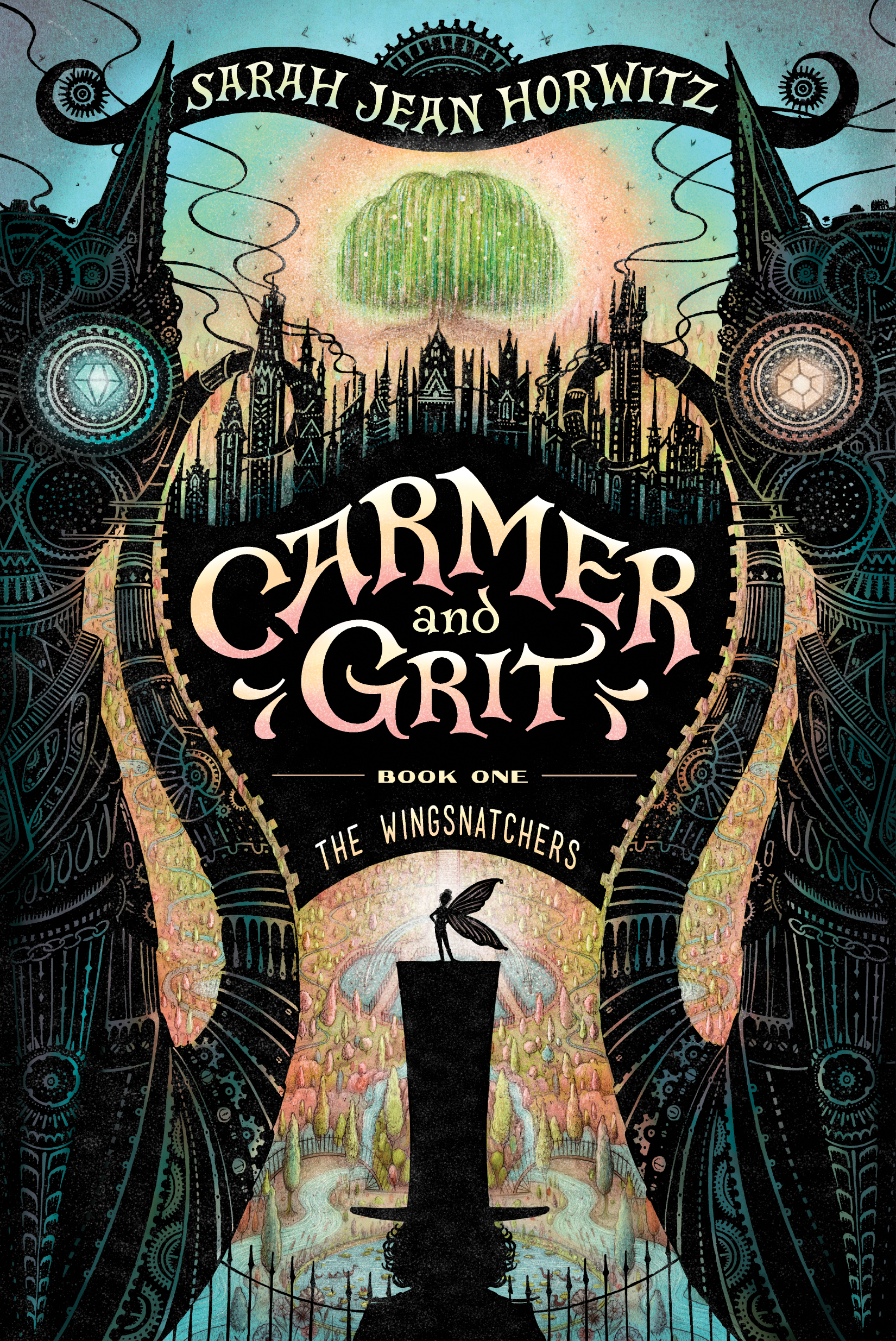The cover of the book "Karma and Grit: Book 1, The Wing Snatchers" by Sarah Jean Horwitz is a highly ornate and whimsical color illustration in portrait orientation. At the top of the cover, the author's name, Sarah Jean Horwitz, is displayed in a black, curvy banner with a wavy, scroll-like design. Below it, a lime green, weeping willow tree glows with a pink hue against a peach background.

Dominating the center is the book's title, "Karma and Grit," in bold, hand-drawn, whimsical orange text, with "Book 1, The Wing Snatchers" written below in smaller letters in an arc. Flanking the title are two mechanical Siamese cats facing each other, adding to the fantastical elements of the cover.

Toward the bottom, a silhouette of a man wearing an extremely tall black top hat stands out. Perched on top of the hat is a small winged fairy, also in silhouette. The background is a vibrant, colorful forest with predominantly red trees, interspersed with green ones, and a cityscape featuring Gothic structures, creating a magical and captivating scene.

The edges of the cover are decorated with intricate black designs, including curved, tentacle-like features with illuminating eyes — one aqua and the other peach. Overall, the cover's detailed and whimsical artwork sets a fantastical tone for the story within.